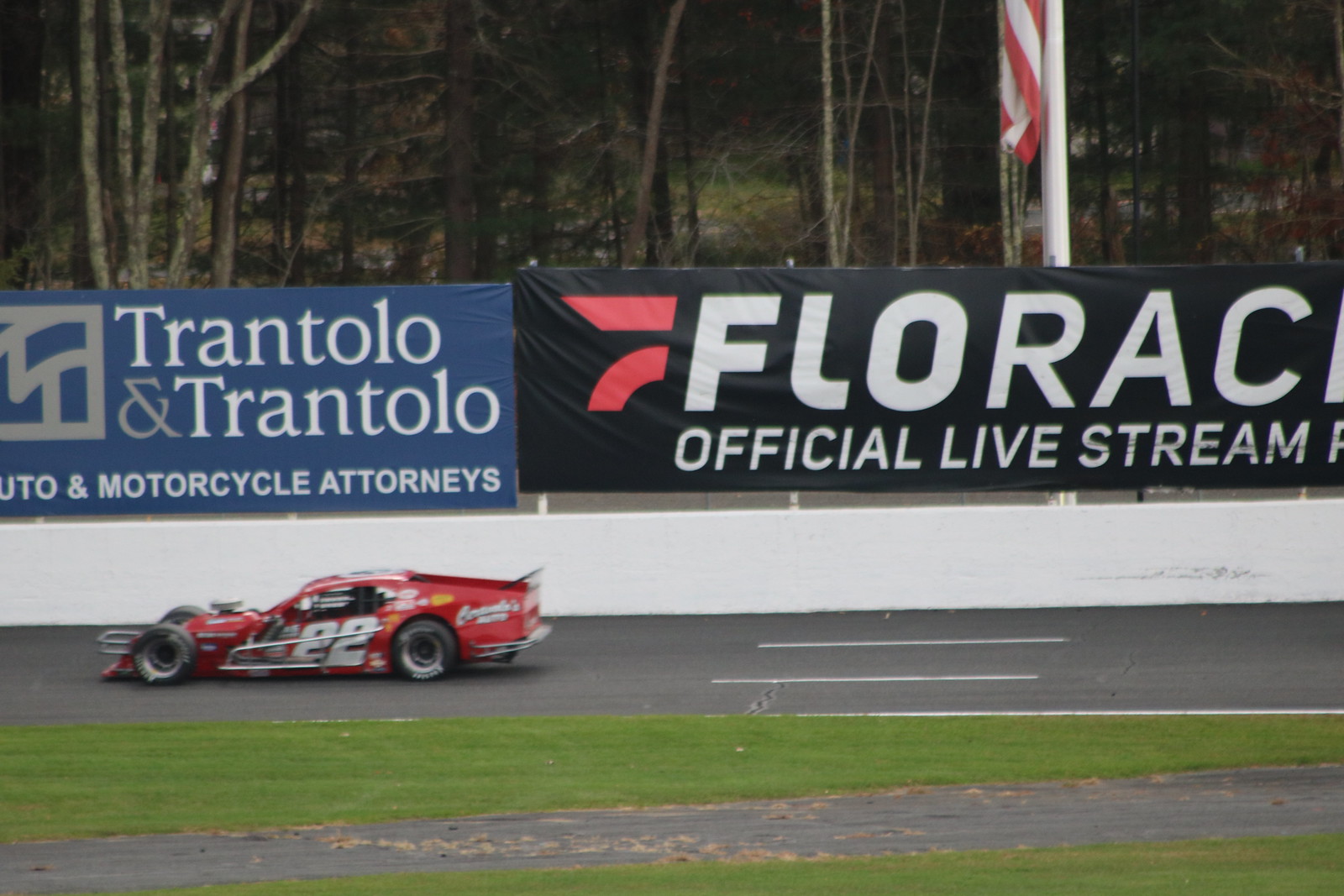This photograph captures the dynamic scene of a red race car, numbered 22, speeding along a race track, creating a blurred effect indicative of its high velocity. The car, with black tires and the number painted in white, races on a black or gray track marked by white hash lines. Inside the track, there is a green grassy area, while the outside is bordered by a white stem wall. Above this wall, two prominent advertising banners are displayed: one for "Trantolo and Trantolo, Auto and Motorcycle Attorneys," featuring a blue background and white text, and the other for "FLORAC Official Livestream," with white text on a black background, although part of the text is cut off. The backdrop is filled with a wooded area and partial view of an American flag, showing red and white stripes, indicating the photo's daytime setting. There is a notable absence of people or an audience, drawing full attention to the car in motion.